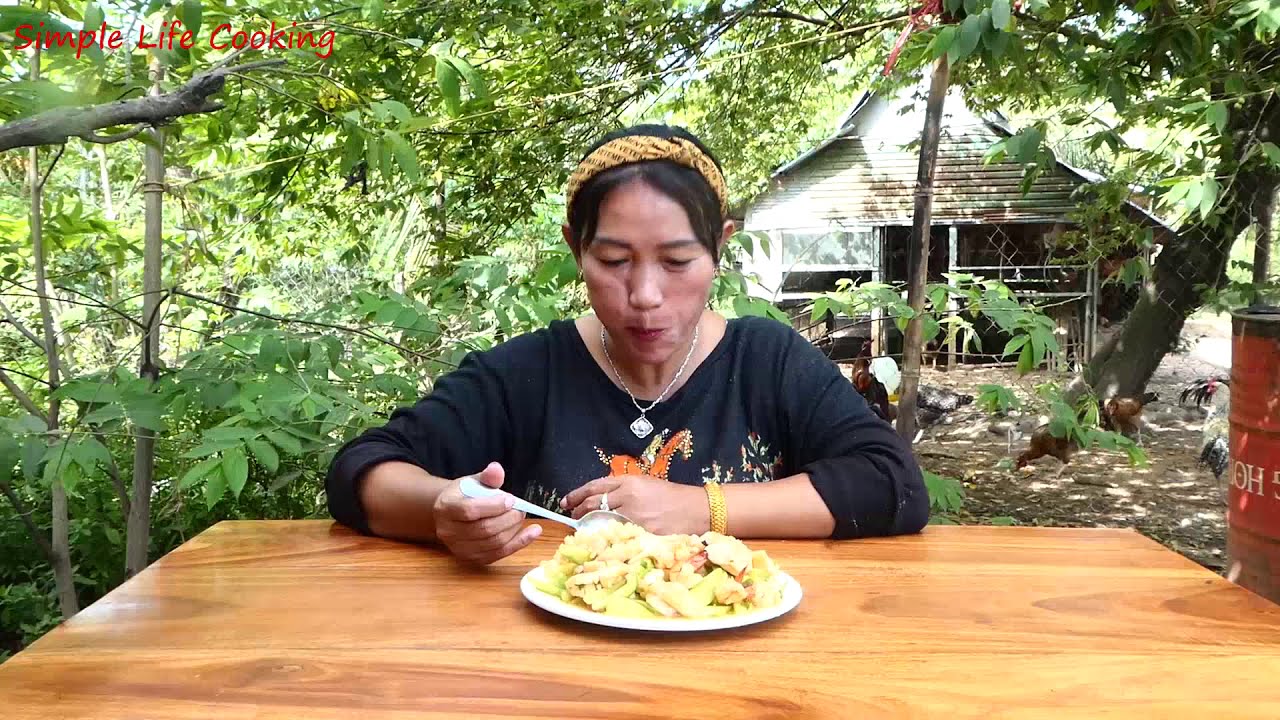In a rustic outdoor setting, a woman in her 50s is seated at a small wooden table, mid-chew with a mouthful of food. She's dressed in a black long-sleeve shirt adorned with a print of flowers and a person on a horse, a yellow and black headband, and a necklace with a square pendant. In front of her is a white plate piled high with a mix of possibly vegetables, chicken, and seafood, featuring yellow, white, and green tones. She holds a spoon in one hand, while her other hand rests on the table. To her right, the edge of a red barrel is visible. The background reveals a backyard or field, with trees, leaves, and perhaps some chickens and a duck near the barrel. In the upper left corner, in thin red font, are the words "Simple Life Cooking." Further back, a rustic shack made of wood or bamboo stands, partially obscured by the natural surroundings.